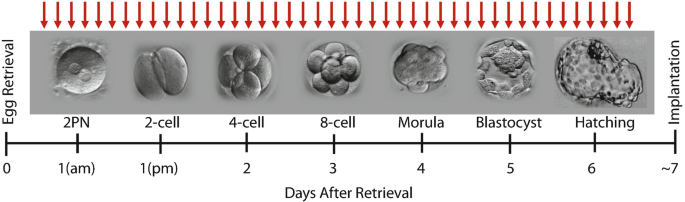The image is a detailed timeline chart illustrating the stages of cell division following egg retrieval, from left to right. On the left side, it is labeled "Egg Retrieval," and the bottom axis, marked "Days After Retrieval" in black text, is numbered from 0 to 1 a.m., 1 p.m., 2 p.m., 3 p.m., 4 p.m., 5 p.m., 6 p.m., and 7 p.m. Each time marker corresponds to a specific stage of cellular development, illustrated with seven microscopic images. These images are annotated sequentially: at 1 a.m. it says "2 p.m.," at 1 p.m. it shows a "2-cell" stage, followed by "4-cell" at 2 p.m., "8-cell" at 3 p.m., "morula" at 4 p.m., "blastocyst" at 5 p.m., and "hatching" at 6 p.m., culminating in "implantation" at 7 p.m. The top section of the chart features numerous red arrows pointing downward at each image. The images depict rapid cell division and development, likely of an organism that grows quickly, suggesting it may not be a human.